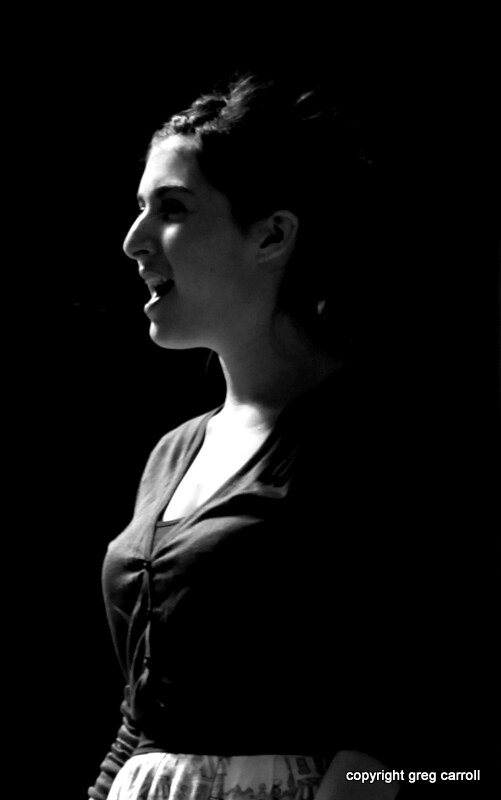This black and white photograph captures a young woman in the midst of a performance or rehearsal, likely on a stage. The atmosphere is dramatic, with a completely black background that makes her dark attire blend in, save for the spotlight illuminating her face and neck. She is dressed in a dark blouse, or possibly a cardigan, layered over a discernible black tank top, and appears to pair this with a skirt. Her dark hair, which might be styled with braids at the top, is tied back. The spotlight, presumably from above, highlights her expressive face as she looks to the left, her mouth open as if singing or speaking. The image is credited to Greg Carroll, noted by a white-font watermark in the bottom right corner, reading "Copyright, Greg Carroll."